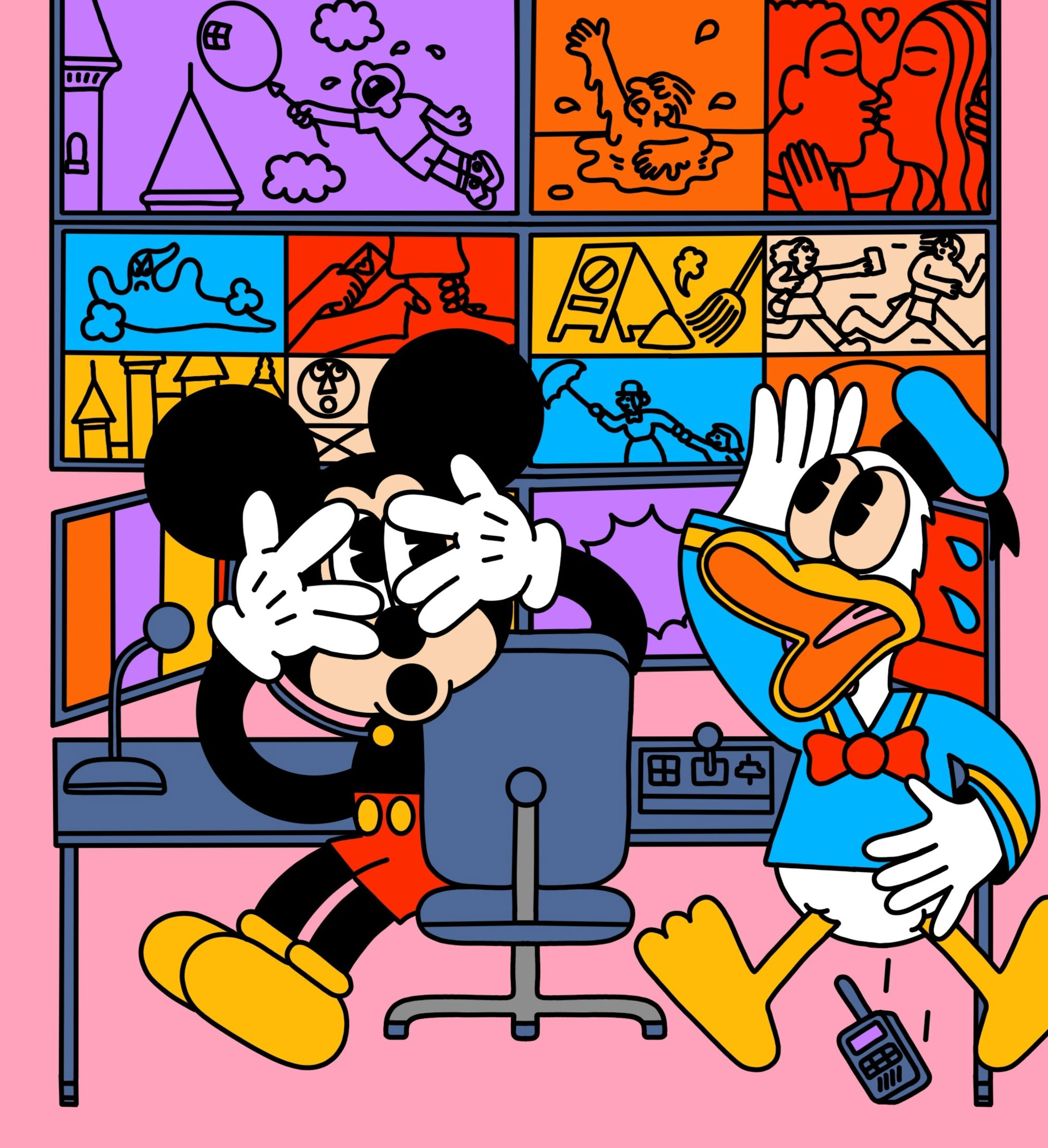In this detailed pixel art illustration, the cartoon characters Mickey Mouse and Donald Duck from Disney are depicted inside a room, with a distinctly pink background. Mickey Mouse, recognizable with his black body, red shorts with golden buttons, white gloves, and yellow shoes, is seated sideways in a rolling office chair. He appears to be playing peekaboo with his hands, his fingers spread open wide over his surprised, open-mouthed face. In front of him, there is a desk adorned with a microphone, some electronic control devices, and several computer monitors. Behind Mickey, the wall features a display with various colorful pixelated images, including scenes of a person flying with a balloon, someone drowning in water, two people kissing, another person cleaning, a baby holding her mother's hand under an umbrella, and a person running after another.

To Mickey’s right stands Donald Duck, also expressing astonishment. Dressed in his signature blue shirt with yellow stripes, red bow tie, black and blue hat, and white gloves, Donald Duck is portrayed mid-jump with his feet spread apart, his wide-eyed, open-mouthed face turned to the upper left. Next to his face, one hand is raised in shock, while below him on the floor lies a fallen walkie-talkie, presumably dropped from his hand. The scene conveys a sense of surprise and urgency, highlighting the unexpected events displayed on the screens in front of them.